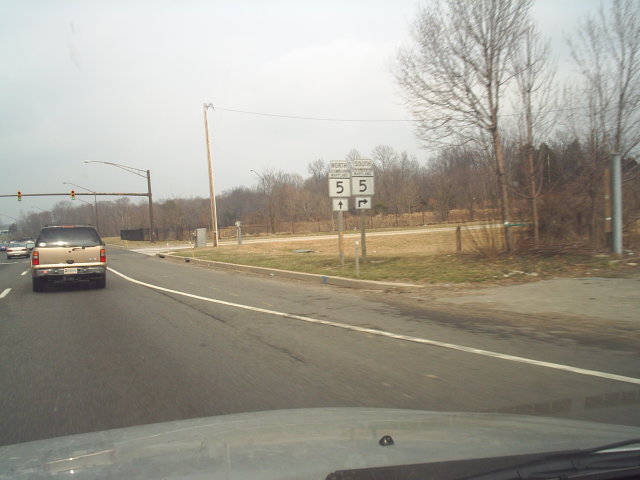The photograph captures a scene from inside a car, looking out across its light blue or gray hood through the front windshield. Central to the image, there's a goldy-brown SUV positioned about 10 meters ahead, without its lights on. The road, which is black with white lane markings, extends forward with overhead traffic lights visible in the distance. Prominently featured are signs for the 5 North and 5 South freeways, alongside a 55 miles per hour speed limit sign, which has arrows pointing both straight ahead and to the right, suggesting directions north and east. To the right side of the road, there's an area of green grass, possibly a trail or sidewalk, accompanied by bare trees and an electrical pole. The style of the image suggests it may have been taken from a dash cam or a head-mounted camera, capturing a traditional driving scene.